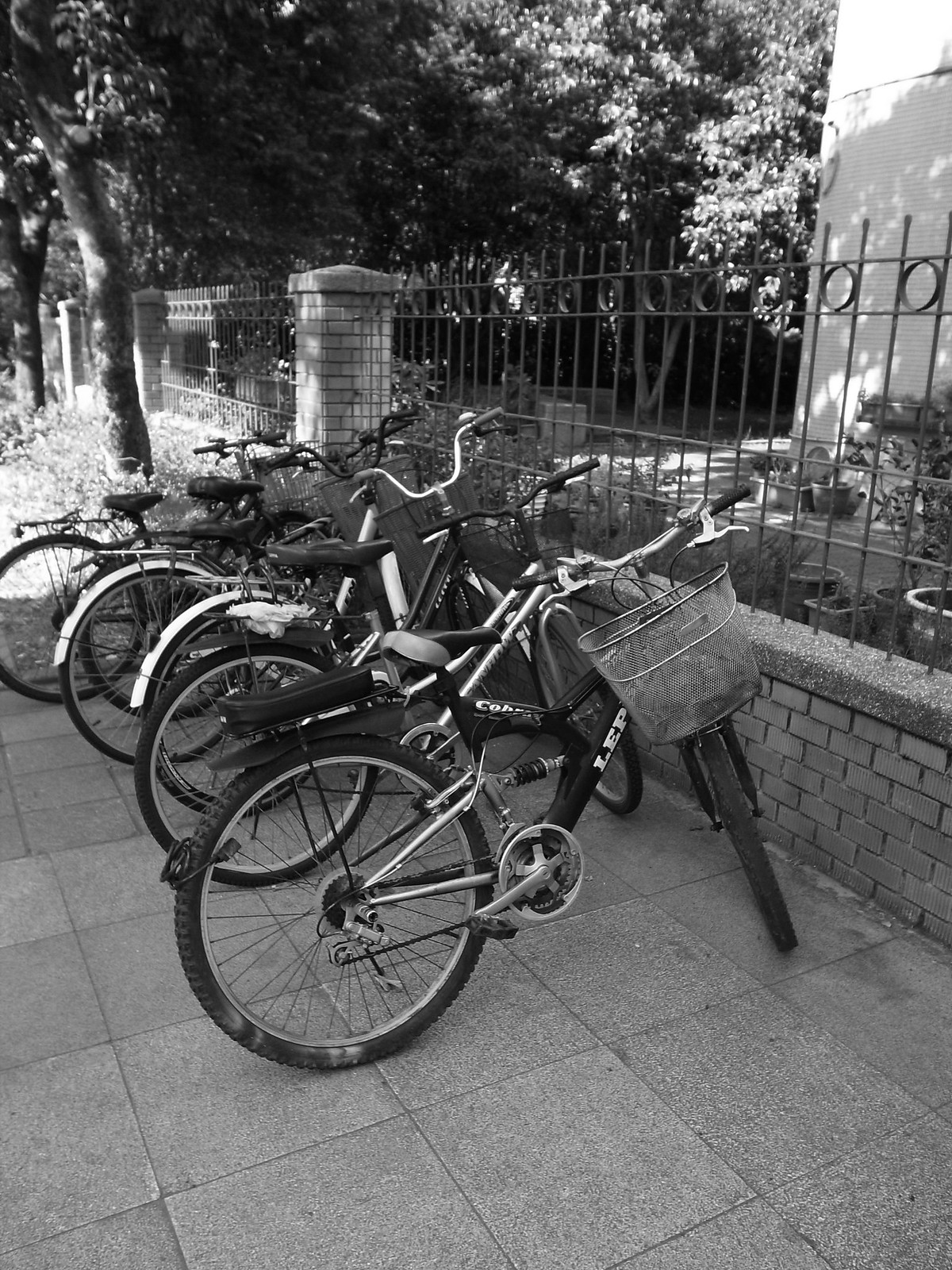This black-and-white photograph captures a serene scene of five vintage bicycles, some equipped with baskets and mudguards, slightly leaning to the left against a weathered stone wall. The pavement beneath the bikes is composed of square concrete tiles. In front of the bicycles, a distinctive fence made of a combination of brick and iron railings stretches along the entire wall. This fence features vertical metal poles with intricate circular decorations and occasional rectangular brick sections with slanted tops. Behind this fence, the wall is dotted with thin metal rods that form part of the fence structure, and beyond that, a lush array of tall trees with expansive canopies provide shade, their leaves stretching over the wall into a courtyard. This courtyard scene reveals potted plants of varying sizes near a stone-lined building visible through the openings in the fence. A line of trees on the left side of the courtyard adds to the idyllic ambiance, lit by sunlight filtering through their branches. The overall daylight atmosphere and details like the bikes' baskets and panniers suggest the setting could be a quiet street or a college campus.